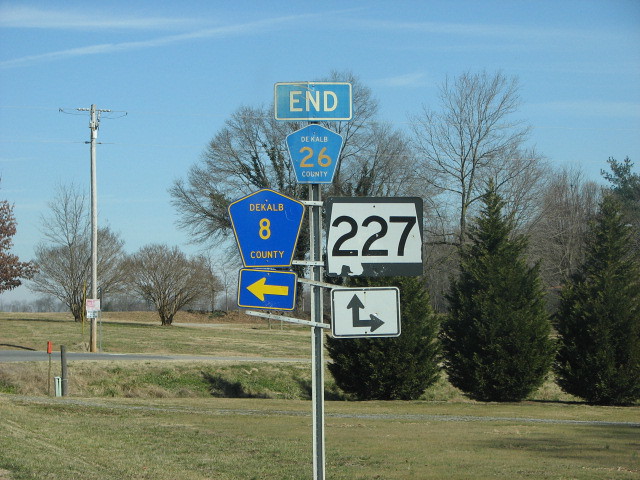This daytime photograph captures a roadside scene with a clear view of various street signs mounted on a metal pole. At the pinnacle of the pole, a rectangular blue sign with white letters reading "END" takes prominence. Directly below it, a shield-shaped sign indicates "DeKalb 26 County." Hanging off the side, on the upper left section of the pole, is another shield-shaped sign displaying "Caleb 8 County." Adjacent to that, on the right, a white and black sign bears the number "227." Beneath the "Caleb 8 County" sign, a blue sign with a yellow left-pointing arrow is visible. Similarly, under the "227" sign, there is an L-shaped double arrow pointing upwards and to the right. The backdrop features a horizontal road and three deciduous shrubs aligned beside each other. Additional foliage and leafless trees populate the landscape in the distance.